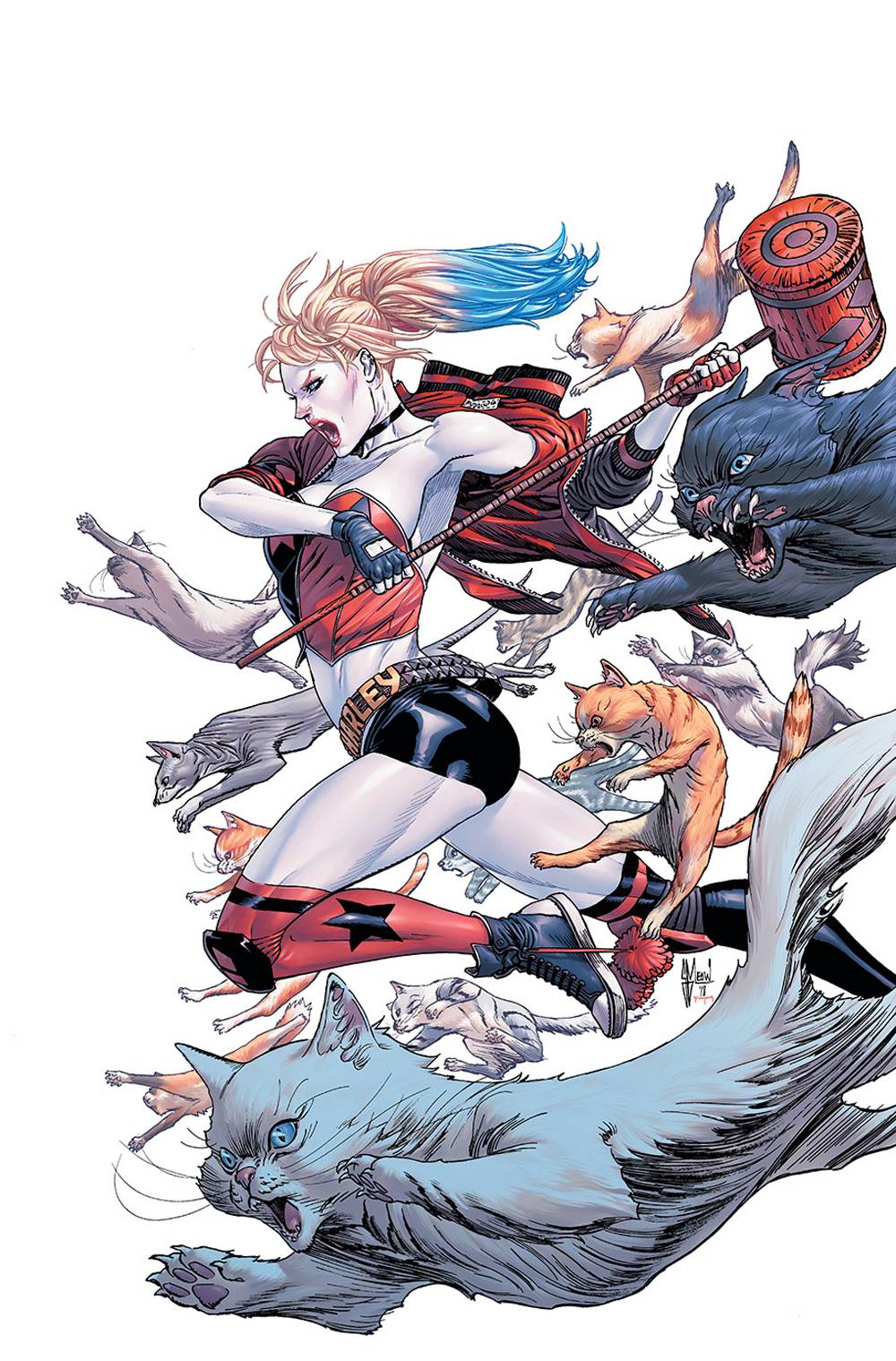In this vibrant digital artwork, we see the iconic fictional character Harley Quinn from the Batman DC universe, dynamically leaping towards the left with one knee bent forward and the other leg extended backward. She sports a red and black halter top, a matching jacket, and very short black shorts with a belt around her waist emblazoned with "Harley." Harley's blonde hair, styled in pigtails, has its tips dyed blue. She wears long, red and black socks paired with blue and white sneakers, and a black knee pad on her forward knee. In her hands, she clutches a large sledgehammer-like mallet with a thin handle, resembling rebar, poised as if about to strike. Surrounding her are about ten fierce-looking cats of various colors, including black, gray, orange, white, and light blue, all mid-pounce with their sharp teeth bared, adding to the chaotic and violent scene. The cats' ferocity mirrors Harley's own intense expression as she attacks an unseen target.